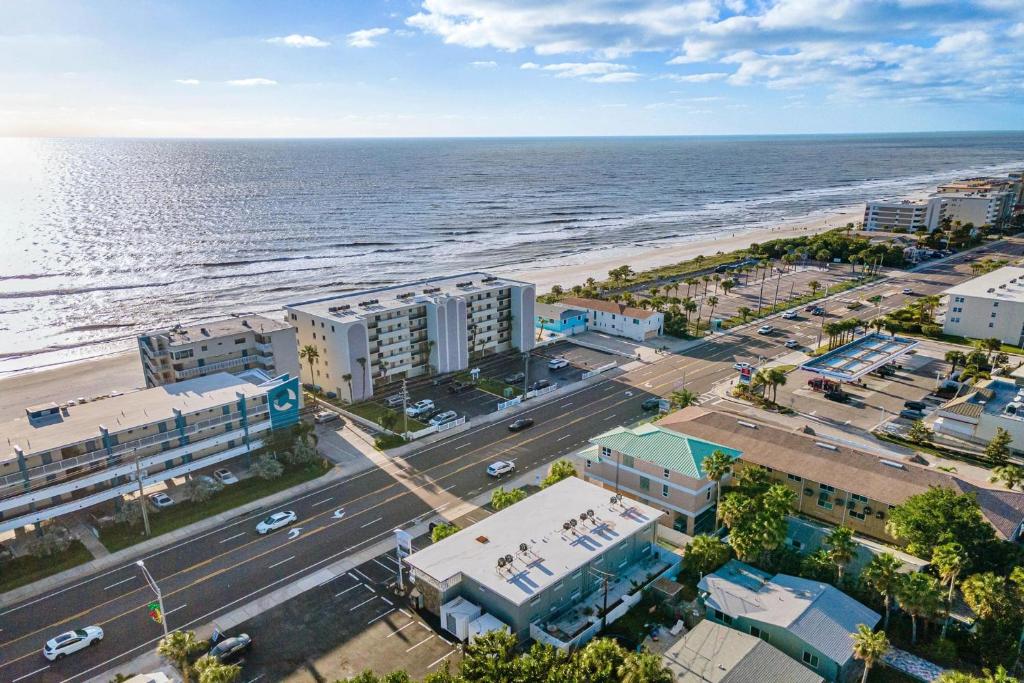This image depicts a detailed bird’s-eye view of a seaside town, with a picturesque blend of natural and urban elements. The top quarter of the photograph showcases a partly cloudy light blue sky overlaying a light grey-blue ocean. Moving downward, the middle section transitions from ocean waves gently meeting a sandy tan beach to a bustling coastal area. 

In the lower half of the image, a series of buildings, including what appear to be condos or apartment complexes, align the waterfront. Scattered amongst these structures are vibrant green patches of palm trees and other tree varieties, adding a touch of nature amidst the urban landscape. A clearly defined four-lane asphalt road, marked with dotted lines and arrows, traverses the area, with cars visible on it.

Towards the bottom left, a more intricate network of residential buildings, possibly houses, stretches upward to the right middle section, interspersed with more trees and a possible gas station. The perspective from above, likely captured via a drone, provides a comprehensive view of roofs, parking lots, and streets meandering between blocks of buildings. The overall scene evokes a sense of an American coastal town, possibly located somewhere in Florida or another similar beachside locale.